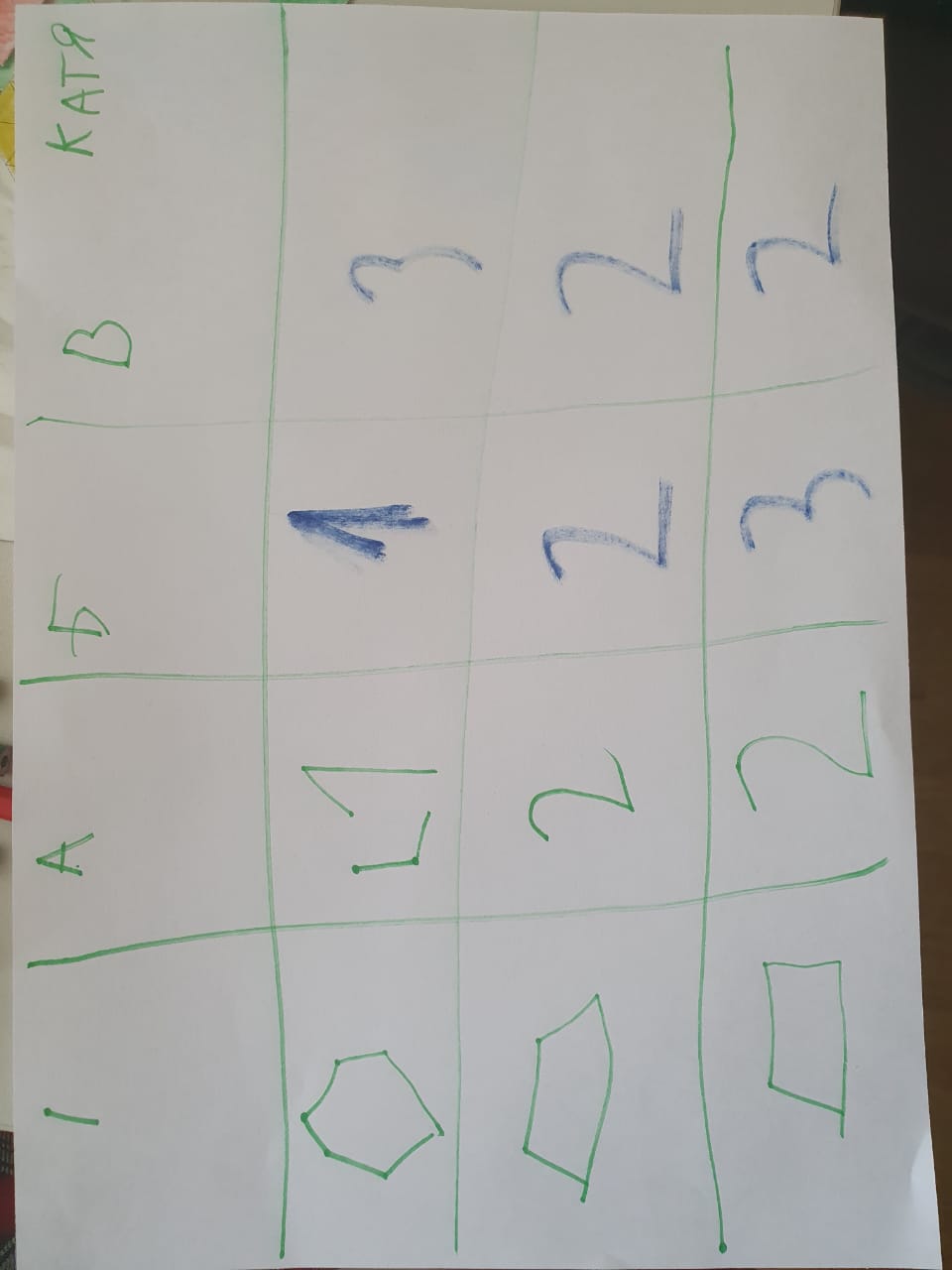This photograph captures a white sheet of paper positioned upright, featuring symbols and childlike handwriting. In the top right corner, the letters "K-A-T-R" are written in green, with the 'R' appearing inversely. A grid of 4x4 fields dominates the paper, each containing a mix of symbols and alphanumeric characters. The grid lines and most content are drawn in green. Within the grid, you can discern letters such as "I," "A," "B," and "L," and numbers like "1," "2," and "3." Interspersed among these are three distinct geometric symbols: a square, an octagon, and a pentagon. Some numbers are faintly sketched in blue marker, adding a subtle contrast. The overall aesthetic suggests a playful and educational purpose.